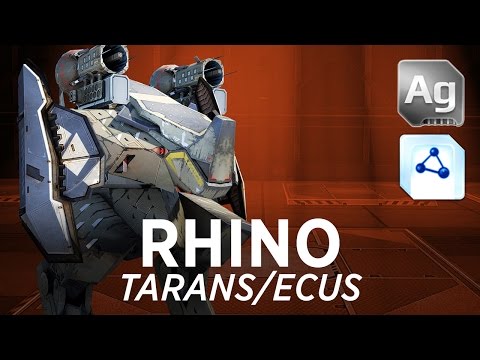The image presents a highly detailed, digitally crafted representation of a futuristic mech suit, fittingly named "Rhino Terrans/ECUS." This imposing bipedal robot, predominantly colored in blue with white and gray accents, stands prominently in the foreground. Its mechanical design evokes the likeness of a rhinoceros, complete with a metallic horn and two large, round cannons positioned on its upper torso. Strikingly modern, the robot features two prominent jet engines on its back, accented with red lines.

The backdrop resembles a high-tech garage, drenched in a red filter that amplifies the industrial ambiance. The metallic flooring is meticulously marked with caution lines, and the surrounding walls reinforce the setting's high-tech aesthetic. Text overlay in white highlights the mech’s name, "Rhino Terrans/ECUS," reinforcing its identity.

To the right side of the image, two distinctive logos are visible. The upper logo, silver in color, displays the letters "AG," referencing silver in the periodic table of elements. Below it, in a light blue box, another emblem features a nuclear design with three blue spheres interconnected by lines, evoking atomic or molecular imagery. This scene might be a promotional piece for a game, a modeling program, or even a concept artwork, radiating a fusion of creativity and advanced robotics.